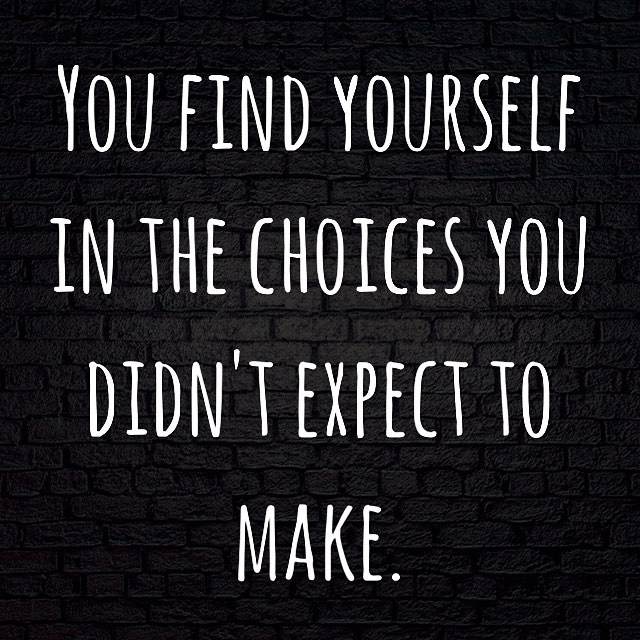The image features a subtle, light-gray brick wall that has been painted black to create a textured, solid black background. Centered on this backdrop is a profound quote in white, all-capital letters, styled to look like a faux handwritten sans-serif font. The text reads: "YOU FIND YOURSELF IN THE CHOICES YOU DIDN'T EXPECT TO MAKE," split across four lines with "MAKE" prominently centered on the fourth line. Despite the minimalist presentation, including slightly crooked letters, the message aims to provide moral support, often found shared on social media. The positioning and simplicity give it a striking yet contemplative effect.